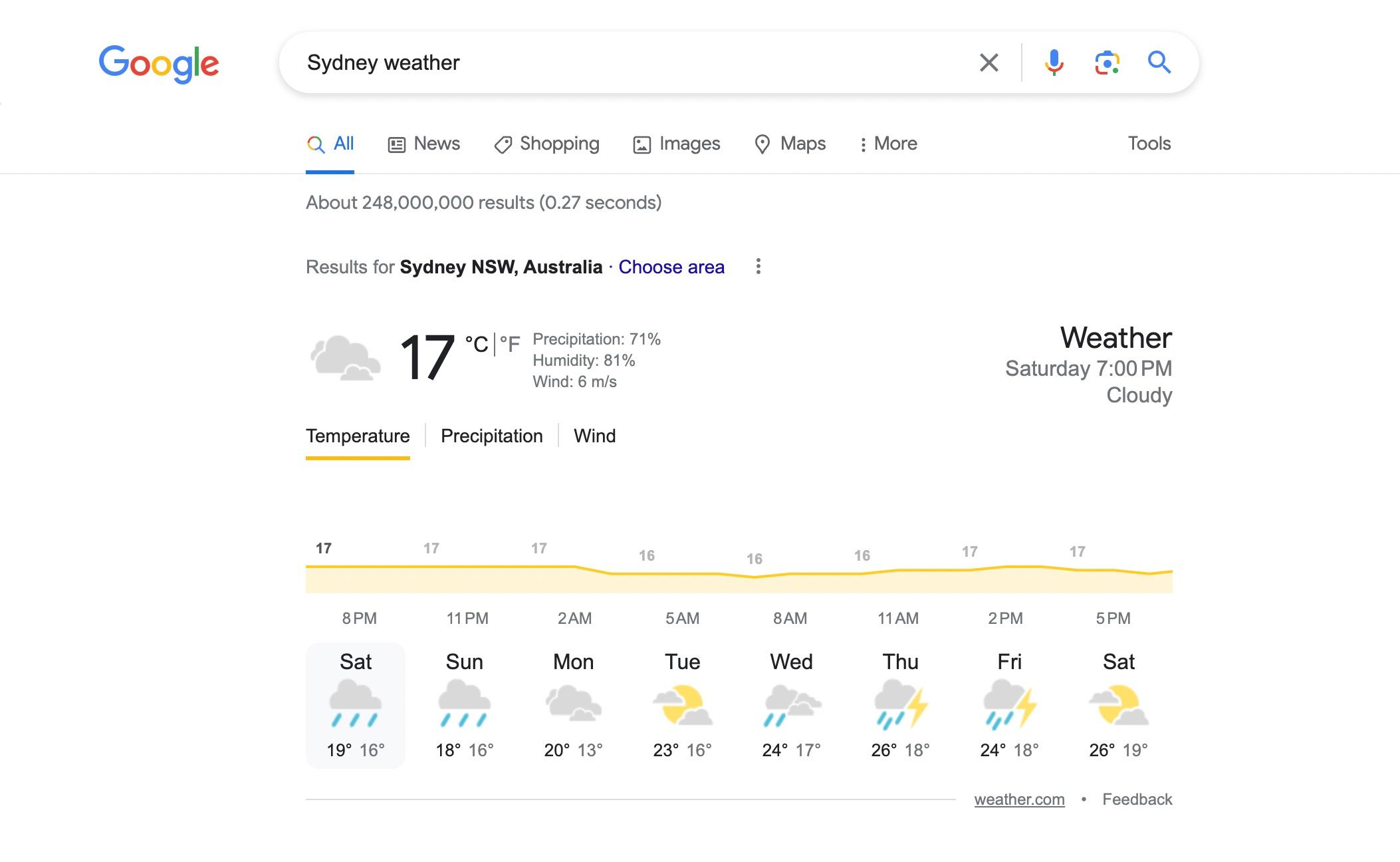This image displays a Google search result detailing the weather forecast for Sydney, New South Wales, Australia. The search query "Sydney weather" is highlighted in a blue box at the top of the screen, accompanied by icons for a microphone, camera, and search. The search returned approximately 248 million results in 27 seconds. 

The weather summary shows a current temperature of 17°C with a gray cloud icon indicating a 71% chance of precipitation, 81% humidity, and winds at 6 km/h. The timestamp is Saturday at 7 p.m., with an additional note of cloudy conditions.

Beneath this summary is a detailed weather forecast presented on a map and timeline. The weekly forecast begins with:
- **Saturday:** Rain, 19°C
- **Sunday:** Rain, 18°C
- **Monday:** Cloudy, 20°C (with updates approximately every three hours)
- **Tuesday:** Partly sunny, partly cloudy, 23°C
- **Wednesday:** Cloudy and rainy, 24°C
- **Thursday:** Cloudy, rainy, with sunshine, 26°C
- **Friday:** Cloudy, rainy, with sunshine, 24°C
- **Following Saturday:** Cloudy and sunny, 26°C, ending at 5 p.m.

Additionally, users have the options to click on detailed views for precipitation and wind conditions.